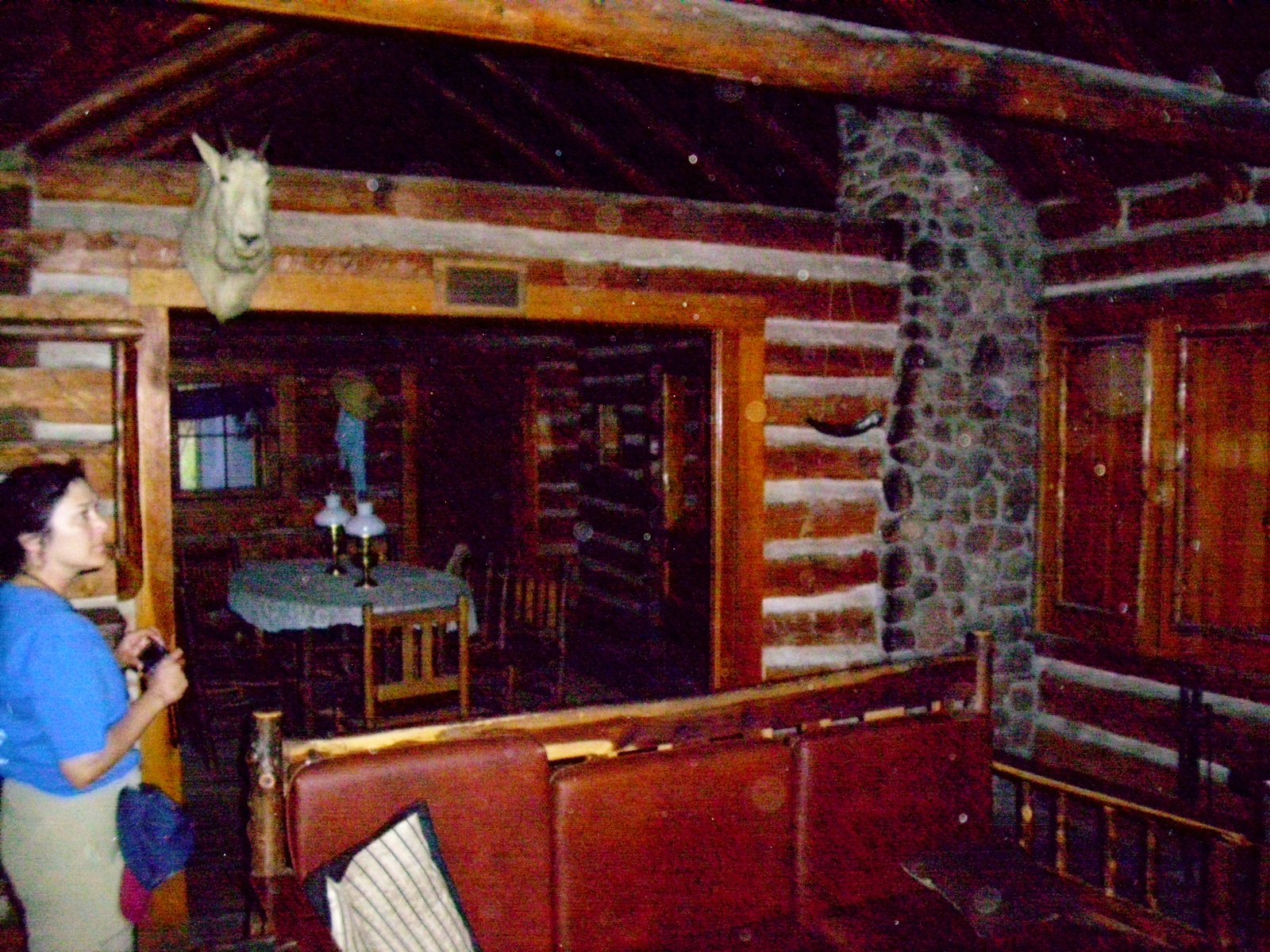In this nostalgic image, a woman wearing a blue shirt and tan-colored pants stands to the lower left side of an old cabin interior. The cabin features wooden walls made of horizontal logs and wooden beams across the ceiling, creating a rustic atmosphere. The furniture, including brown pieces with white cushions, adds to the vintage charm. In the background, a dining table with a white tablecloth and two lamps is surrounded by wooden chairs. Prominently, a stone structure resembling a chimney extends upwards, and a mounted head of a ram or goat hangs on the wall, which initially gives the impression of additional animal figures created by the stone patterning. The woman appears to be observing this intriguing array of textures and decor. A window in the back allows light into the otherwise cozy, wood-clad room, enhancing the overall feel of stepping back in time.